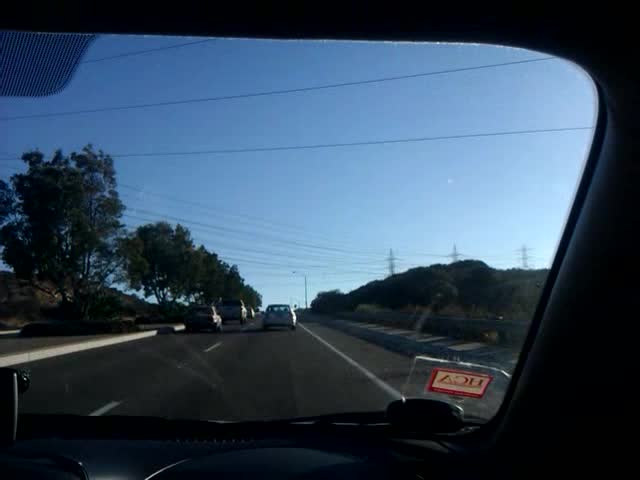The image captures a blue-skied, late afternoon scene from the front passenger seat of a moving car, looking out through the windshield onto a highway. The dark gray road ahead is divided by a dotted white line separating two lanes. A solid white line marks the edge of the right lane, next to which lies a sidewalk bordered by sagebrush and trees. To the left of the car, trees densely line the roadside. Several cars are visible: a silver car directly in front of the viewer in their lane, and three or four cars traveling in the opposite direction. Major power lines stretch across the road in the distance. A red and white rectangular sticker with "HCA" in red is visible in the bottom right corner of the windshield. The highway extends under a clear, cloudless sky dotted with power transmission towers, flanked by hills and trees.